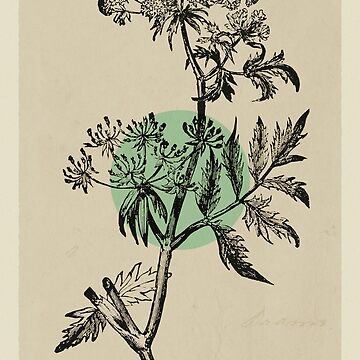The image depicts a detailed pen and ink drawing of a leafy plant against a tan, canvas-like background. The plant, drawn in black, features a stiff, dense stem with branches splitting off, each bearing multiple leaves. Toward the top of the plant, the leaves transition into spidery, tendril-like structures, seemingly reaching upward towards the light. The background includes a muted mint green circle centrally placed behind the plant, contributing a subtle color contrast. The composition is framed by a lighter beige border on the left and right sides, while the top and bottom edges appear deliberately cut off. There is a faint, almost unreadable signature in the bottom right corner, adding an element of authenticity to the artwork, which appears to resemble a woodblock print or painting.